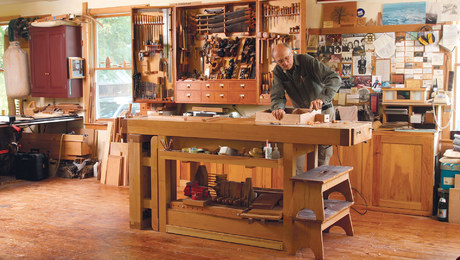In this detailed image of a cluttered woodworker's shop, a man, likely around the age of 60 with short grey hair on the sides and a balding middle, is intensely focused on constructing a wooden box frame. He wears a dark grey long-sleeve shirt paired with grey trousers and glasses, his hands diligently holding the frame together. The large wooden workstation in front of him, brown in color and featuring various compartments to hold his essentials, further emphasizes his dedication to his craft. Scattered tools, wooden pieces, and a stepping stool highlight the bustling, chaotic nature of the workspace. Behind him, a collage of photos, letters, and cards adorns the back wall, adding a personal touch. Wooden shelves and cabinets filled with tools line the background, with a window on the left side showing an overcast day outside.